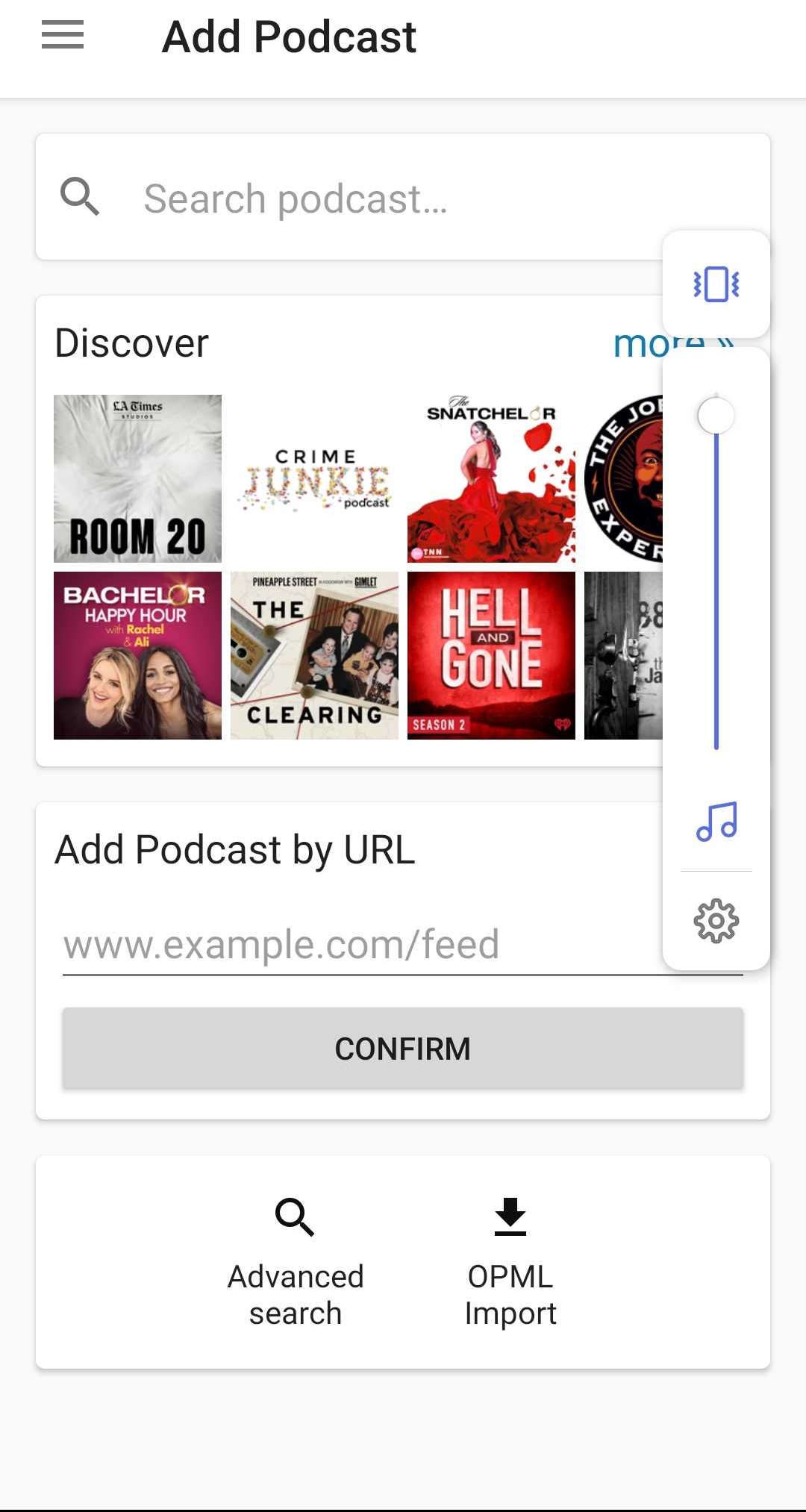The image displays the interface of a podcast app or website. At the top left corner, there is a black-colored hamburger menu icon. Immediately to the right, bold black text reads "Add Podcast." Below this, a search bar labeled "Search Podcast" is stationed, with a magnifying glass icon to its left.

In the central section, a heading titled "Discover" is shown. Below this heading is a grid of square images representing different podcasts. The first image is labeled "Room 20," followed by "Crime Junkie Podcast" next to it. The third image is titled "Naturaler." The fourth image, partially cut off, seemingly represents "The Joe Rogan Experience." 

In the row beneath, the first podcast displayed is "Bachelor Happy Hour with Rachel and Allie," followed by a podcast named "Declaring." Next in line is "Hell and Gone," and the last visible podcast in this row shows only the number "88" in black and white.

Further down, the interface features an "Add Podcast by URL" section, accompanied by an input field to enter the URL. A "Confirm" button is located just below this input field. At the very bottom of the interface, there are two categories labeled "Advanced Search" and "OPML Import."